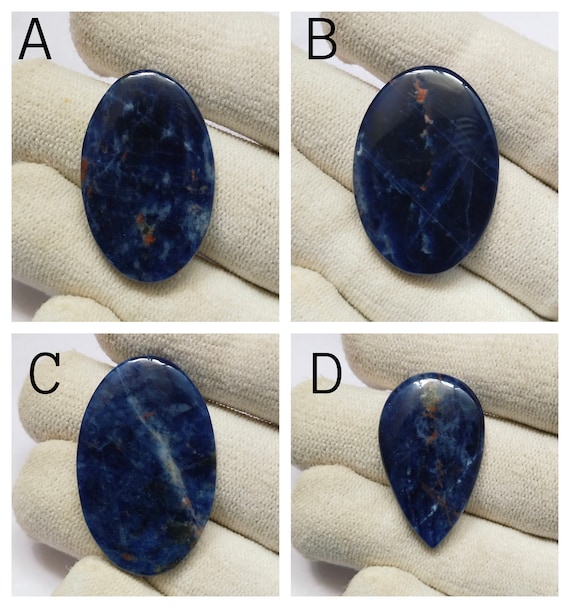This image is a four-part photograph arranged in a grid, with two images on the top row and two on the bottom, labeled A, B, C, and D respectively. Each section features a close-up view of slightly differently-shaped polished gemstones held by a gloved hand wearing a white glove. The gemstones in sections A, B, and C are all predominantly oval, though they vary slightly in their coloration—displaying dark hues with highlights of red, pink, dark blue, and white flecks. The gemstone in section D departs from the purely oval shape, resembling an exclamation point with its pointed bottom. All the backgrounds in these images are dark blue, flecked with light blue and white, giving a textured and random pattern that complements the colors of the stones.